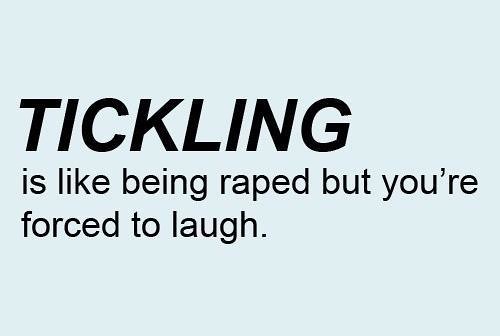The image consists of a small horizontally aligned rectangle with a light bluish-gray background and no border. It prominently features the word "TICKLING" in all caps, bold black letters, left-aligned at the center of the image. Directly below this is a two-line phrase in smaller, standard black text that reads, "it's like being raped, but you're forced to laugh." The background is a solid, very light icy blue color, enhancing the contrast with the black text. There are no images or additional elements; the simplicity of the layout draws attention to the stark and provocative message presented.